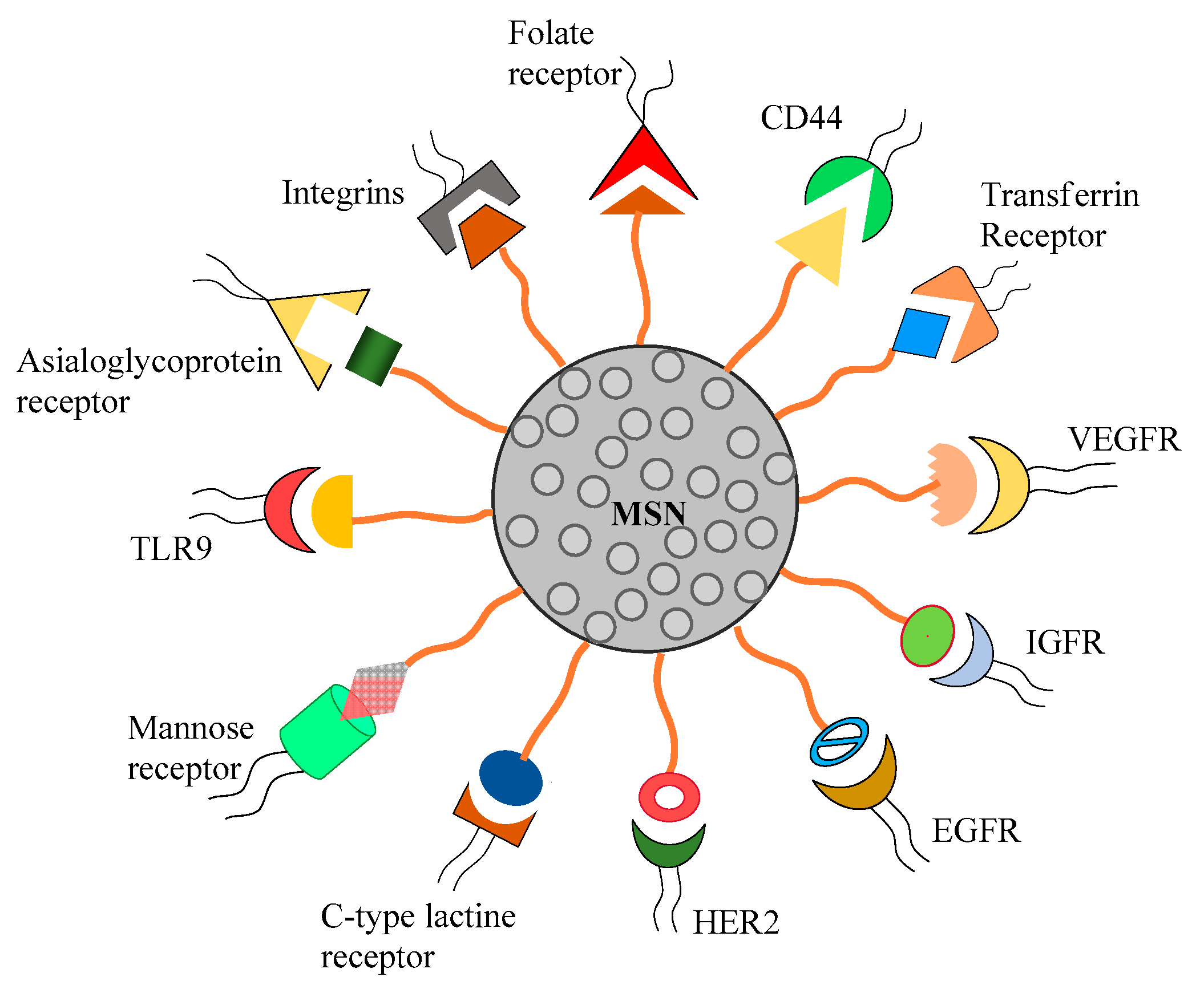The image is a detailed, color-coded biological diagram set against a white background. At the center, there is a gray circle outlined in black, filled with lighter gray circles, and labeled "MSN" in black text. Radiating outward from the central circle are orange lines that lead to various colorful geometric shapes, each paired with a black text label identifying specific receptors and molecular structures. Key labels and shapes include: 
- At the top, an orange line leads to a red triangle labeled "Folate Receptor."
- To the right, another line connects to a label "CD44," which includes a green shape and a yellow triangle.
- Other labeled structures around the central circle include "Transferrin Receptor" with an orange partial square and a blue diamond, "VEGFR" with a yellow half moon and an orange half circle, "HER2" with a green half moon and a red circle, "C-type Lactin Receptor" with a brown half square and a blue oval, and "Mannose Receptor" with a green cylinder and a red diamond, among others.

Additional receptor labels include "IGFR," "EGFR," "TLR9," "ASIALOGLYCOPROTEIN Receptor," and "INTEGRINS," each connected to the central MSN circle with their respective unique geometric shapes and colors. The diagram comprehensively illustrates various receptor types and their connections in a visually organized manner.